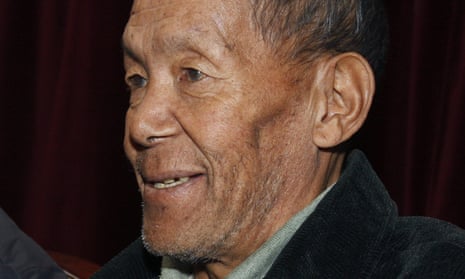The image features a close-up of an elderly Asian man, likely in his 60s or 70s, with a weathered appearance and high cheekbones. His dark, bony face is marked with visible wrinkles, especially on his forehead and around his eyes, and he has very sparse eyebrows. His hair is thin and black, particularly noticeable on the sides of his head. He sports a bit of pure, sparse stubble on his chin. The man is smiling slightly, as if he was speaking moments ago, and is staring straight ahead with a gentle, thoughtful expression. He’s dressed in a black jacket over what appears to be a grayish-green shirt with a gray collar peeking out. The background is a dark, earthy brown with dark red curtains, putting the focus entirely on his face.